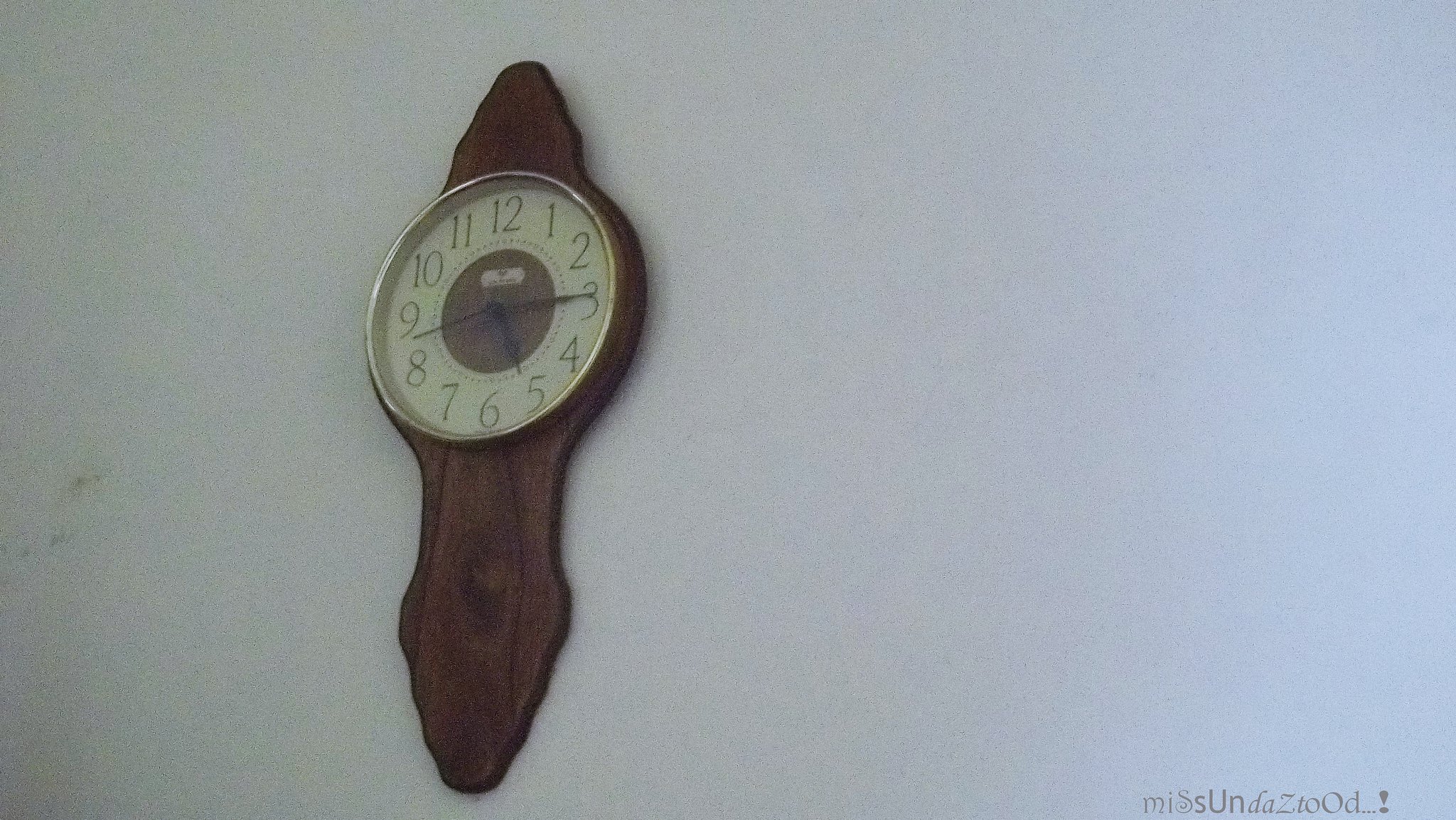This image depicts a wall-mounted clock with a circular face encased in a sleek silver border. The clock face is white and features bold Arabic numerals from 1 to 12, marking each hour around the perimeter. The clock has three hands: a minute hand, an hour hand, and a second hand, which collectively indicate the current time to be approximately 5:15 and 43 seconds. At the center of the clock face, where the hands are anchored, there is an additional brown circular element that adds a touch of contrast to the design.